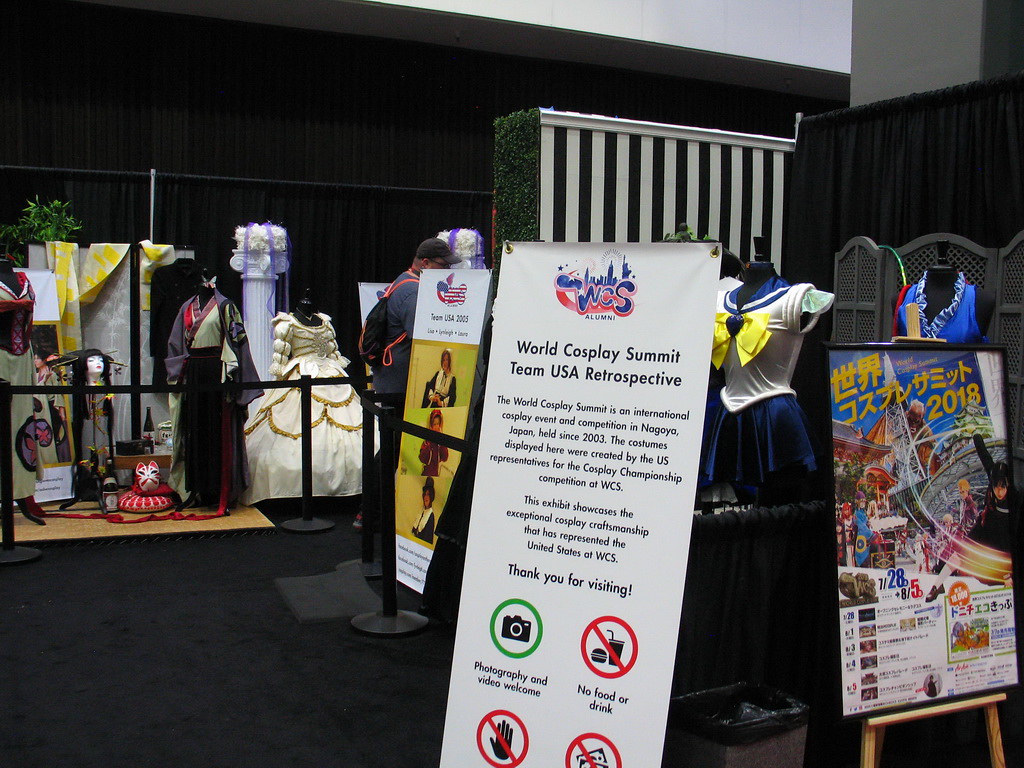This detailed photograph captures an indoor exhibit from the World Cosplay Summit Team USA Retrospective event. The room features long black curtains hanging from gray walls and a dark gray carpet. Centered in the display are several meticulously crafted costumes exhibited on mannequins, each representing different eras and styles. Notably, one costume includes a white blouse with a blue neckline, another is a lavish gold Edwardian-era dress, and yet another features a suit with a purple stripe. Among the costumes, the display context is underlined by a prominent white banner with the headline "WCS Alumni" in blue print with a red outline, followed by "World Cosplay Summit, Team USA Retrospective" in black print. The signage indicates that the World Cosplay Summit is an international cosplay event held in Nagoya, Japan, since 2003, showcasing the exceptional craftsmanship of U.S. representatives. The exhibit invites photography and video, as signified by a green circle with a camera, but prohibits food, drink, and other unspecified activities indicated by red circles with slashes. Additional signage reiterates these rules and provides a warm thank-you to visitors for attending. In the backdrop, further embellishing the scene, is a poster with Asian script except for the year 2018, and a person can be spotted standing discreetly behind one of the displays.